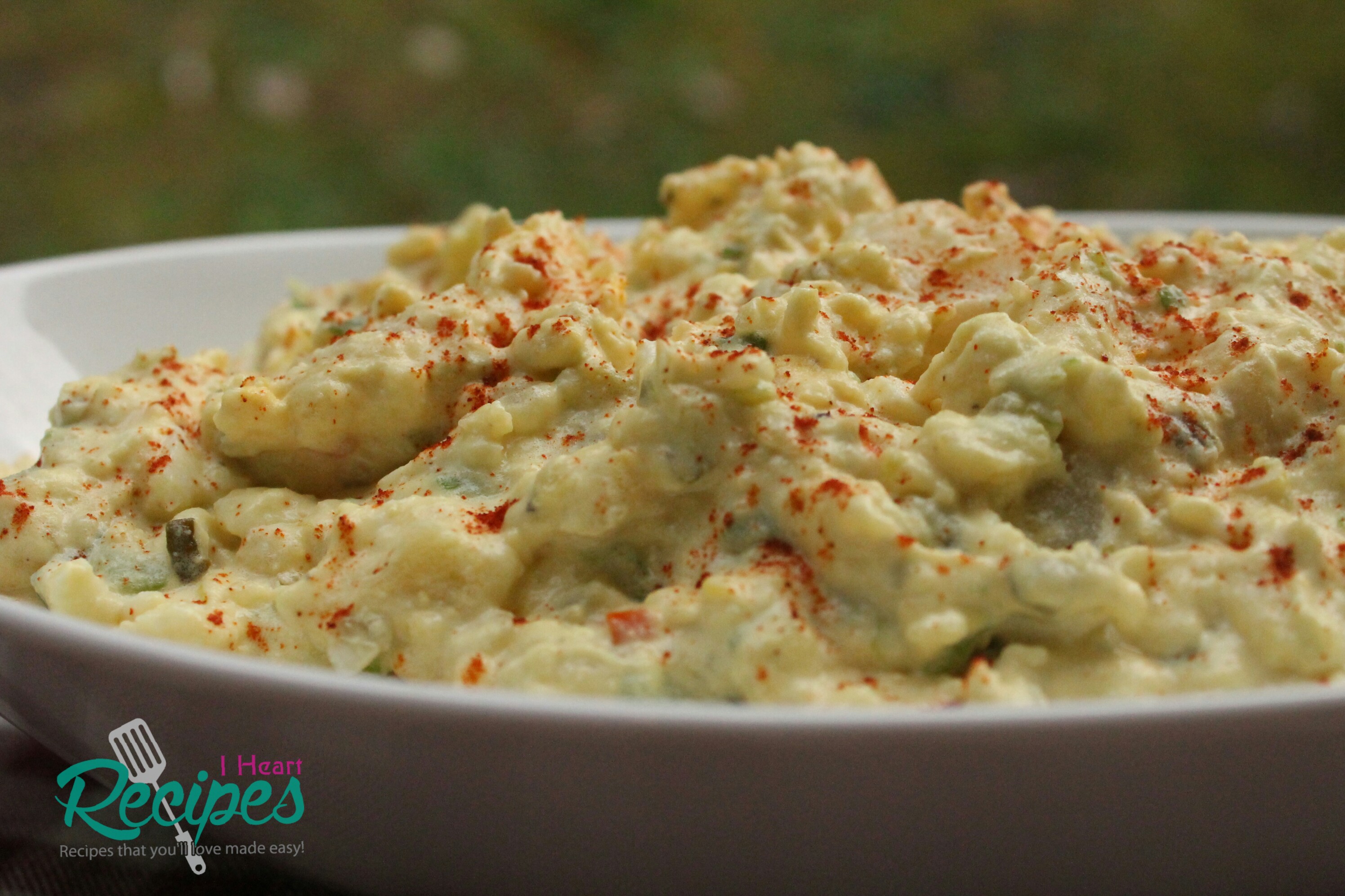In this detailed image, we see a close-up of a white bowl filled with what appears to be potato salad, prominently positioned in the center. The potato salad contains visible chunks of diced potatoes, egg yolks, and egg whites, and is generously garnished with a sprinkling of orange paprika. This colorful dish features signature yellow tones from the potatoes and eggs, accented by green hues, likely from relish. 

In the bottom left corner of the image, the logo "I heart recipes" is displayed, with "I heart" in vibrant pink and "recipes" in teal green. The design incorporates a white spatula that diagonally traverses the text. Beneath the logo, it reads "recipes that you love made easy" in white font. 

The background is deliberately blurred, showing a blend of green shades that suggest grass, adding a contextual hint of an outdoor setting, possibly a picnic. The focus remains sharply on the bowl of potato salad and the accompanying logo in the lower left-hand corner.